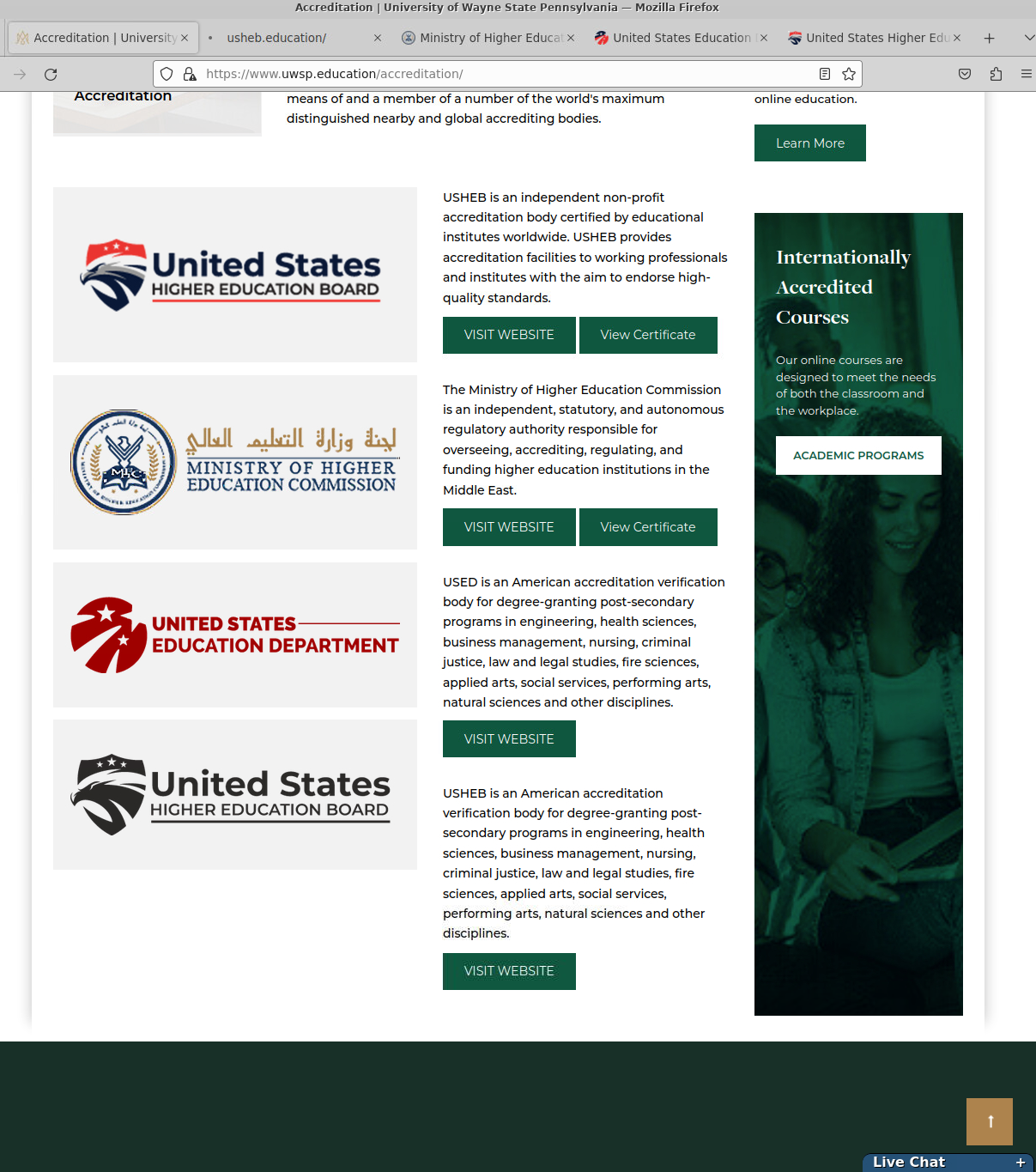The image depicts a browser window opened in Firefox with multiple tabs visible at the top. The active tab is displaying the accreditation page for Wayne State University, Pennsylvania. The tabs extend from the left to the right, indicating several open sessions.

The central focus of the webpage is the authority and details of several educational accreditation bodies. The primary section showcases four different entities related to higher education accreditation. 

1. **United States Higher Education Board:**
   - A badge featuring a bald eagle with red, white, and blue accents.
   - Described as an independent, non-profit accreditation body certified by educational institutions worldwide.
   - Provides options to visit their website or view their certification for legitimacy.

2. **Ministry of Higher Education Commission:**
   - Displays a bald eagle perched on a book.
   - Includes a descriptive statement to the right, a link to their website, and an option to view their certification.

3. **United States Education Department:**
   - Similar structure to the previous entries but only includes a website link without the certification option.

4. **United States Higher Education:**
   - Like the previous entry, it only provides a website link without an option for certification.

Additionally, a live chat feature is noticeable at the bottom right corner of the webpage, available for any immediate inquiries or assistance. The search bar at the top indicates the URL "uwsp.edu/accreditation".